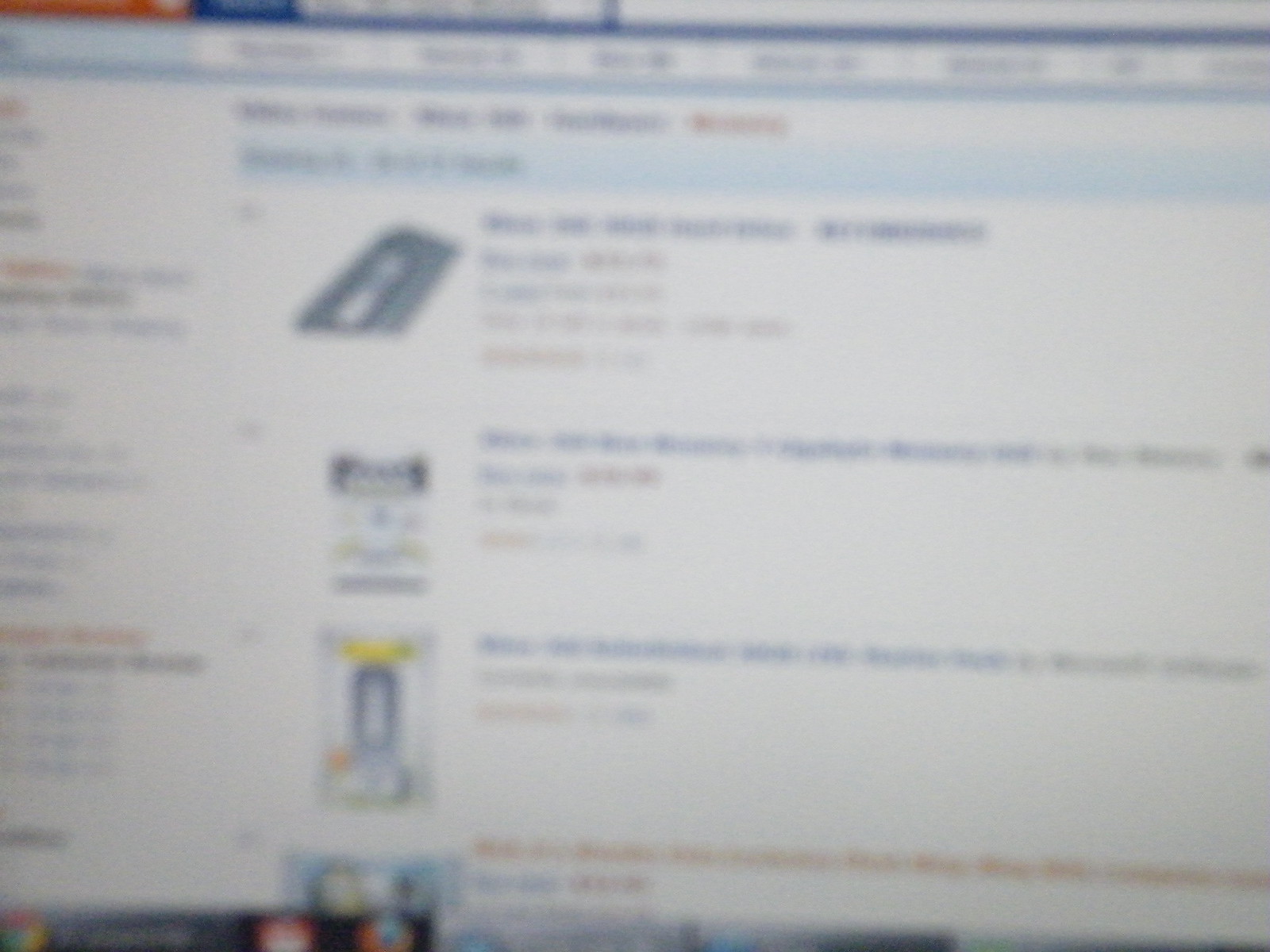The image depicts a very blurry close-up photograph of a computer screen displaying a shopping website, possibly Amazon. The screen shows four rectangular items listed vertically, each with blurry images on the left and unreadable text on the right, which likely describes the products. The website's interface has a white background with orange and blue hues visible at the top left corner. To the left of the product listings, there are various filters for refining search results, such as price and quality options. The bottom portion of the screen features a strip of indistinct colors, including gray and circular red and orange-blue elements. Despite the poor image quality, the layout and details are suggestive of an online catalog or e-commerce site.